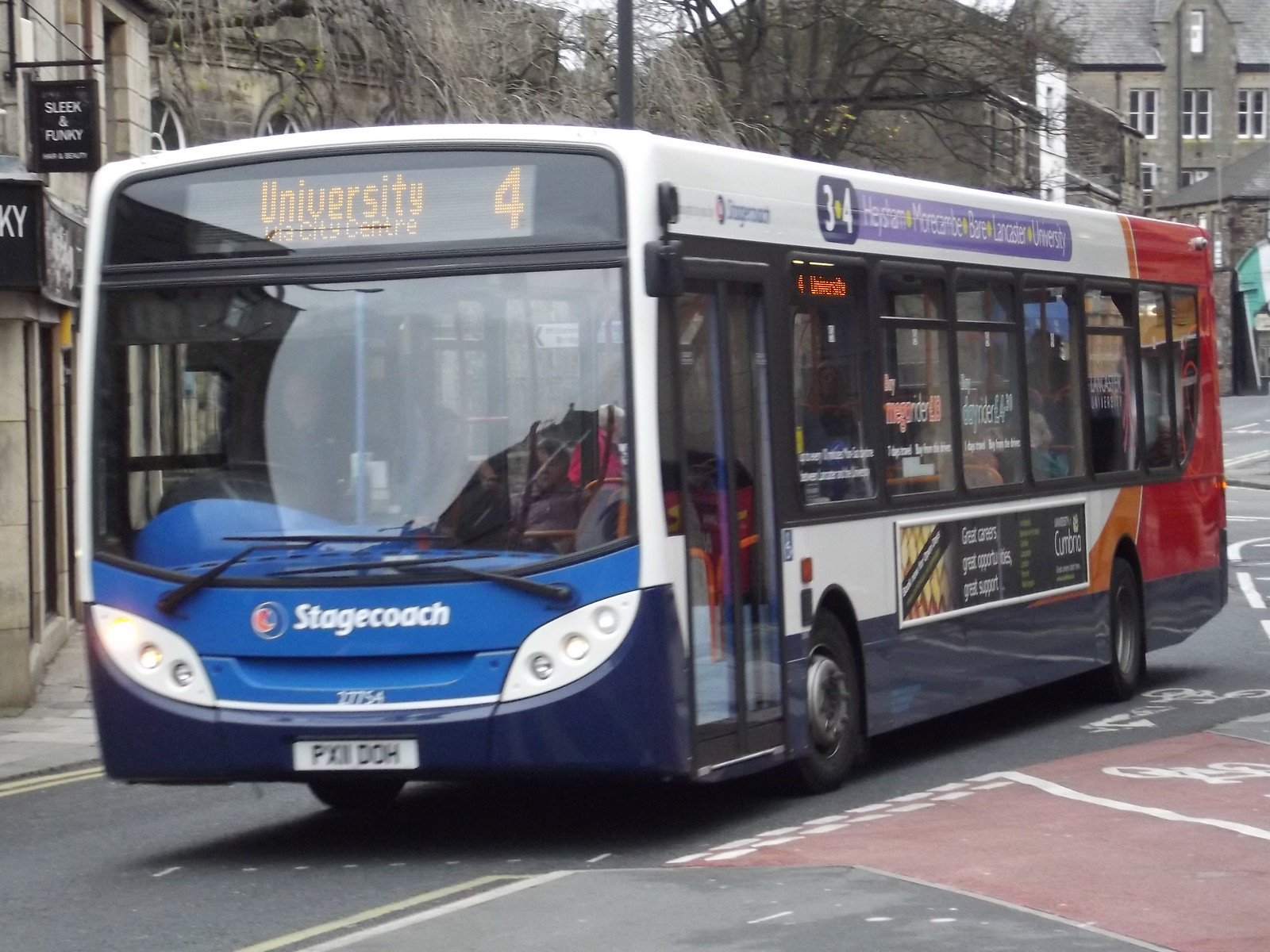The image showcases a modern public transportation bus in the UK, bearing the Stagecoach logo on the front. Its electronic front signage indicates it is the University via City Center route, bus number 4. The bus has a striking design with a white top section, a purple bottom, and red trim towards the rear, along with a swooping orange and red graphic that extends up towards the roof. Several advertisements adorn the side and windows of the bus. Above the windows, multiple city destinations, including Bexar and Lancaster, are listed. The bus is driving along a city street with one lane and a bike lane. The background reveals business signs, including ones for Sleek and Touque, likely suggesting a location in England. Inside, one passenger is visible, indicating the bus is either early in its route or near its end.